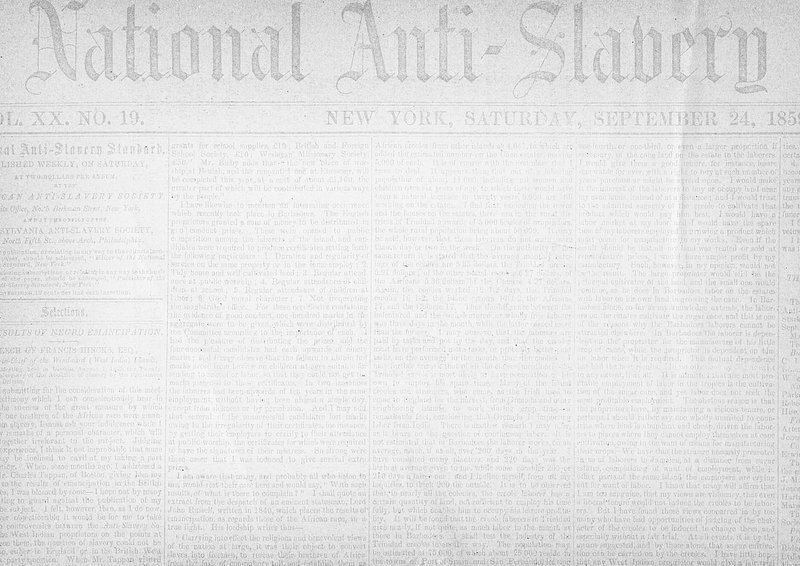This image depicts a photocopy of a faded, grayscale newspaper titled "National Anti-Slavery." The newspaper is identified as Volume XX, Number 19, and was published in New York on Saturday, September 24, 1850, though some of the date detail is unclear. The text is largely illegible due to the poor quality of the scan and the washed-out appearance of the paper, which lacks any pictures. The headline "National Anti-Slavery" is prominently displayed in bold, with subsequent subheadings also bold but smaller. The article is partitioned into five sections below the main heading, although the precise content of the paragraphs is indiscernible due to the faded print. The overall appearance of the newspaper suggests that it is a clean, possibly photocopied extract rather than the original, given its uniform whiteness and absence of any typical age-related discoloration or marks.